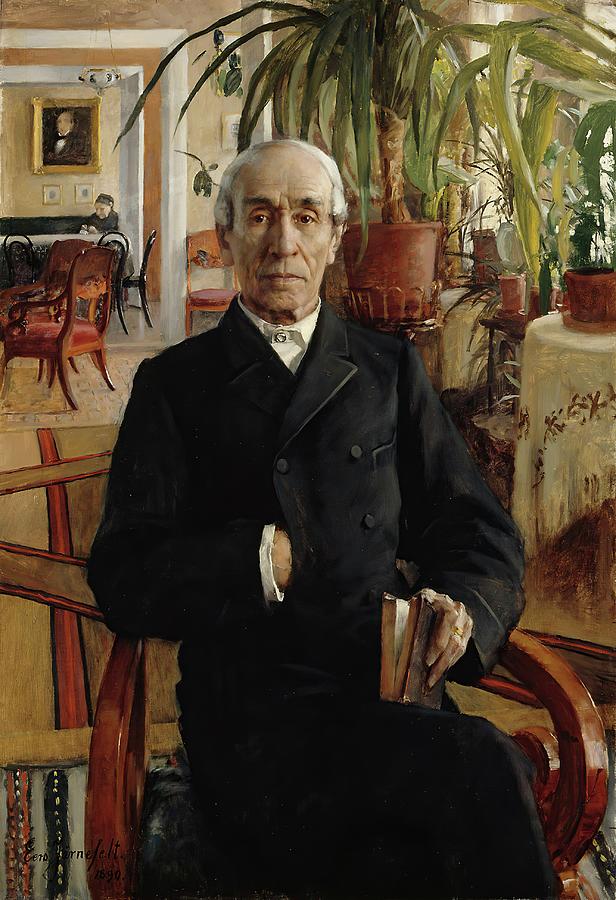This painting, titled "Johann Philipp Palmin" and dating back to circa 1890, is an oil on canvas masterpiece rendered in muted tones of beige, rust, brown, and green. It intricately depicts an old man, presumably Johann Philipp Palmin, seated in an opulent lounge adorned with red velvet upholstered chairs and gold-framed pictures on the walls. The setting is filled with numerous plants and tables, giving the impression of a lush, decorative environment. The central figure, an elderly gentleman with slightly balding, salt-and-pepper hair, commands attention with his intense gaze and weathered, lined face. Dressed in a long, black double-breasted coat, buttoned across, and a white collared shirt, he strikes a stoic, Napoleonic pose with his right hand tucked inside his coat, while his left hand holds a partially open brown book, his finger inserted as if pausing mid-read. A wedding band glints on his finger, adding a personal touch to his distinguished appearance. Behind him, more elements of the lush setting — including a table with a cloth, additional chairs, and an archway with a portrait of another figure — further enrich the scene, making it a vivid and detailed portrait that captures not only the likeness but also the aura of its subject.